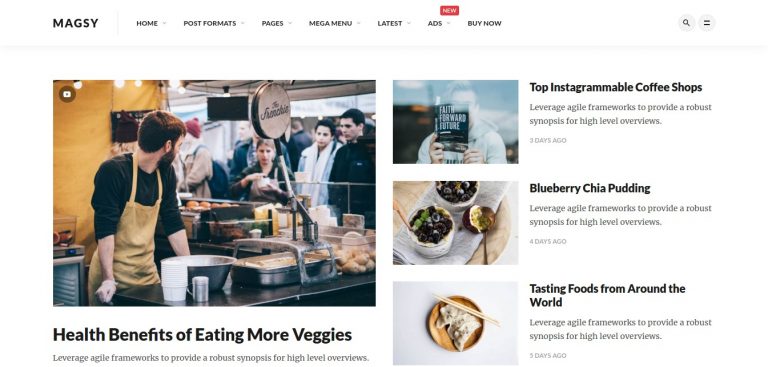This screenshot captures the homepage of a website titled "MagZ," prominently displayed in the upper left corner. The website features a navigation bar at the top with several clickable options, including "Home," "Post Format," "Pages," "Mega Menu," "Latest," "Ads," and "Buy Now." At the top right corner, there is a magnifying glass icon for search functionality and a menu icon represented by two lines within a circle.

The main content area showcases several articles, each accompanied by visuals. The largest article, positioned on the left side, is titled "Health Benefits of Eating More Veggies," and features an image of a quaint bakery scene. The description beneath the title reads, "Leverage agile frameworks to provide a robust synopsis for high-level overviews."

On the right side, three smaller articles are arranged vertically:
1. The top article is titled "Top Instagramable Coffee Shops" and includes an image of a man reading a book. Its description is identical to the main article: "Leverage agile frameworks to provide a robust synopsis for high-level overviews."
2. The middle article is titled "Blueberry Chia Pudding," also accompanied by a generic description: "Leverage agile frameworks to provide a robust synopsis for high-level overviews."
3. The bottom article, "Tasting Foods from Around the World," follows suit with the same description text and imagery format.

Overall, the screenshot provides a glimpse into the visually rich and organized layout of the MagZ homepage, spotlighting various culinary and lifestyle topics.